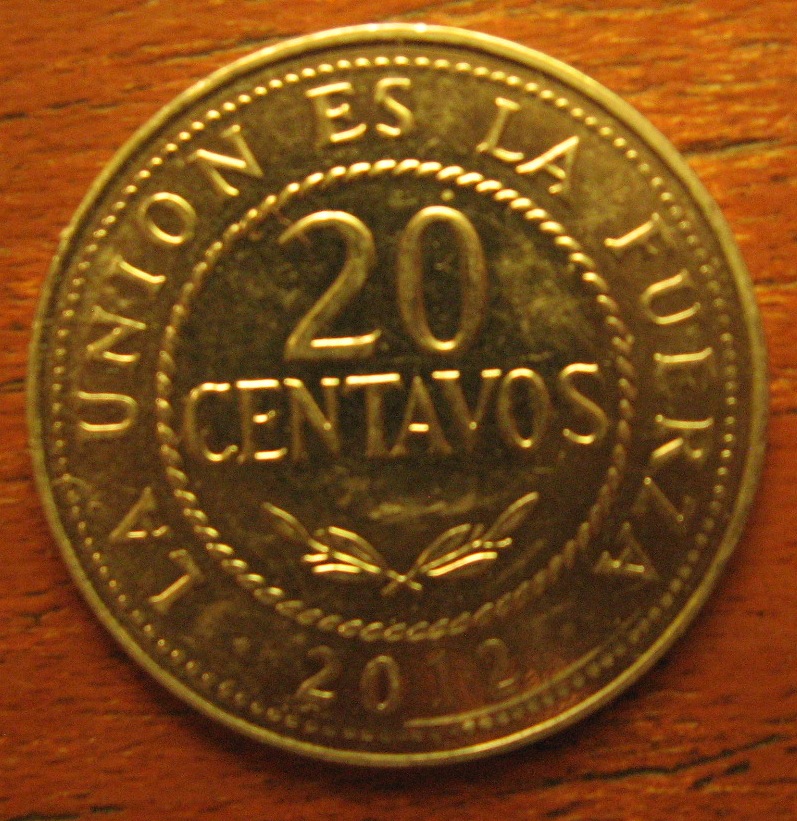The image depicts a close-up of a coin with a golden-tinted appearance, possibly made of or coated with gold. The coin is positioned on a reddish-brown wooden surface and nearly fills the entire square frame of the photograph, with just a hint of the table visible around the edges. The coin is circular and prominently features the denomination "20 Centavos" in the center, flanked below by an intricate design resembling leaves or wheat. Encircling the central inscription is a detailed, rope-like border, followed by an outer ring of small dots forming another circle. Around the top edge of the coin, the inscription "UNIÓN ES LA FUERZA" is imprinted, starting from around the nine o'clock position, along with the year "2012" and the letters "L.A." The coin has a textured, rugged appearance with multiple layered circular designs and borders, giving it a detailed and ornate look.